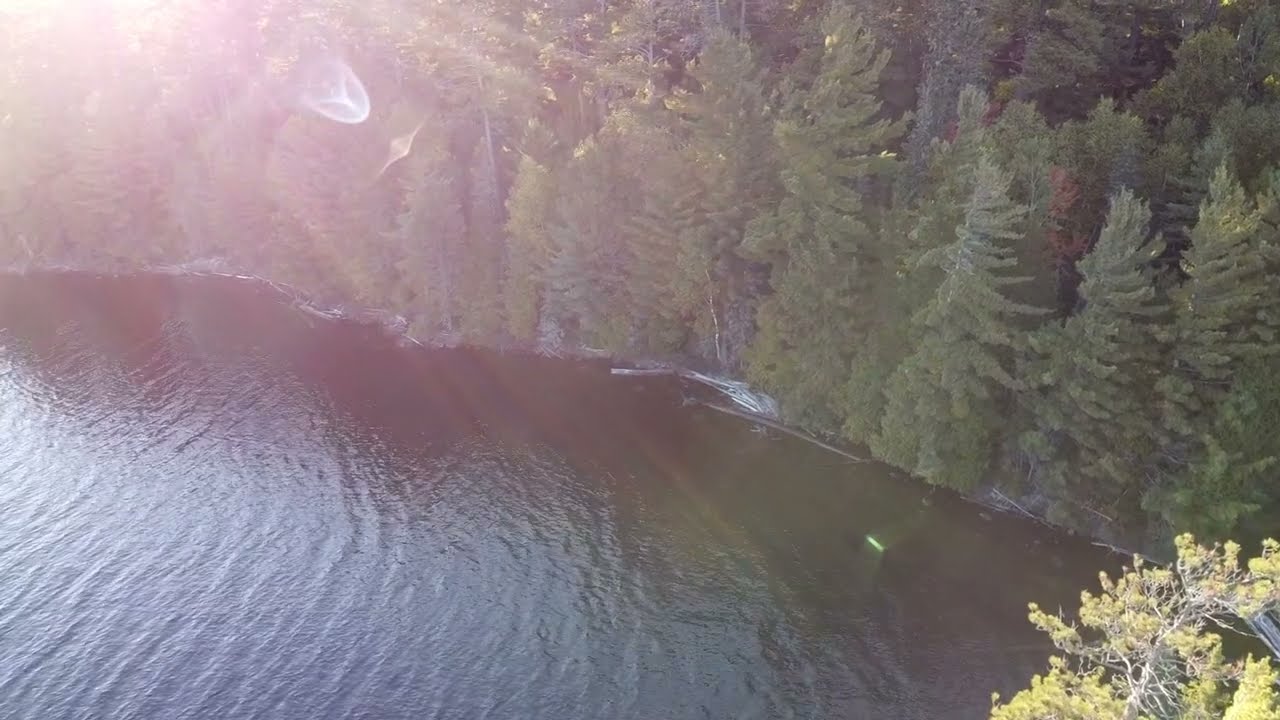The horizontally aligned rectangular image presents an aerial view of a serene pond or lake at the bottom half, with the water appearing brown to dark grayish with gentle ripples. A notable glare from the Sun on the bottom left enhances the reflective quality of the water. Dominating the upper half of the image is a dense forest of tall pine or evergreen trees, extending towards the horizon, emphasizing the wooded nature of the area. The Sun, positioned in the upper left-hand corner, casts bright rays through the trees, creating a stark contrast with the relatively dim right portion. Near the bottom right, a smaller tree with yellowish-green leaves interrupts the expanse of water and the tall pines, adding a touch of color diversity. The overall scene is uninhabited, free from any people, boats, or text, highlighting the natural beauty and tranquility of the landscape.